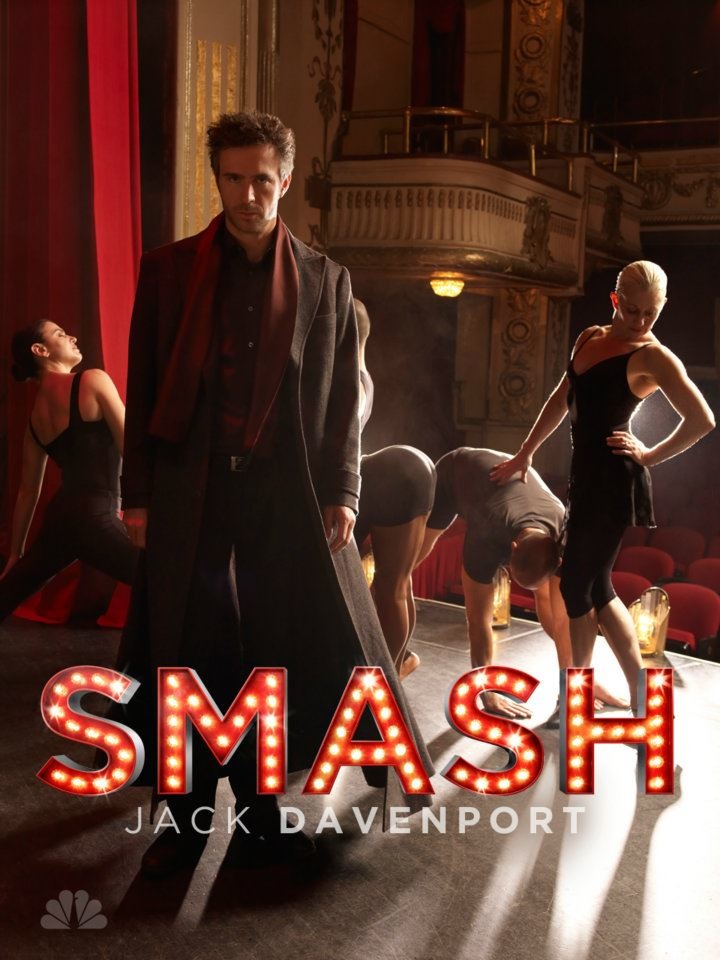The promotional poster for the NBC TV show "Smash" features a dramatic, theater-inspired setting. Dominating the visual is the logo "SMASH" in bold, red, Broadway marquee-style letters adorned with light bulbs, capturing the essence of stage glamour. Beneath the logo is the name "Jack Davenport" in white lettering. The scene is set in a richly detailed theater, complete with old-fashioned balconies, ornate carvings, and ambient lighting that creates an evocative atmosphere.

In the foreground stands a mysterious man with an intense gaze, wearing a long grayish-brown trench coat and a burgundy scarf over a dark shirt. His spiked hair and light beard add to his enigmatic presence. Surrounding him are several ballet dancers dressed in black leotards; a young woman with blonde hair pulled back, and male dancers caught mid-movement in dynamic poses. The carefully arranged lighting, including spotlights and amber hues, enhances the sense of drama and captures the essence of a theatrical performance. The NBC peacock logo is subtly placed in the bottom left-hand corner, anchoring the image as an official promotional material for the network.